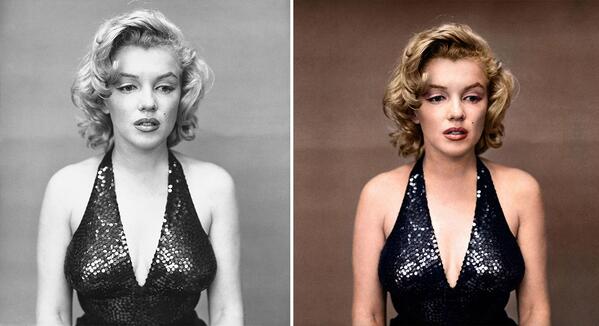The image is a side-by-side comparison of Marilyn Monroe, featuring both a black and white original and a colorized version. On the left, the black and white photograph captures Marilyn in her trademark look: curled blonde hair, a prominent facial mole, and her iconic black sequined dress with a deep neckline. She wears her usual makeup and gazes downward, exuding a melancholic aura. On the right, the same image has been meticulously colorized, giving her skin a white tone with a hint of warmth. Her lips are painted a bronze-red, her eyebrows are brown, and she wears subtle pale pink eyeshadow. The backdrop has been filled in with a brown hue, though it’s unclear if this matches the original setting. The colorized version maintains the same somber expression, emphasizing the emotional depth of the moment captured in the black and white original.